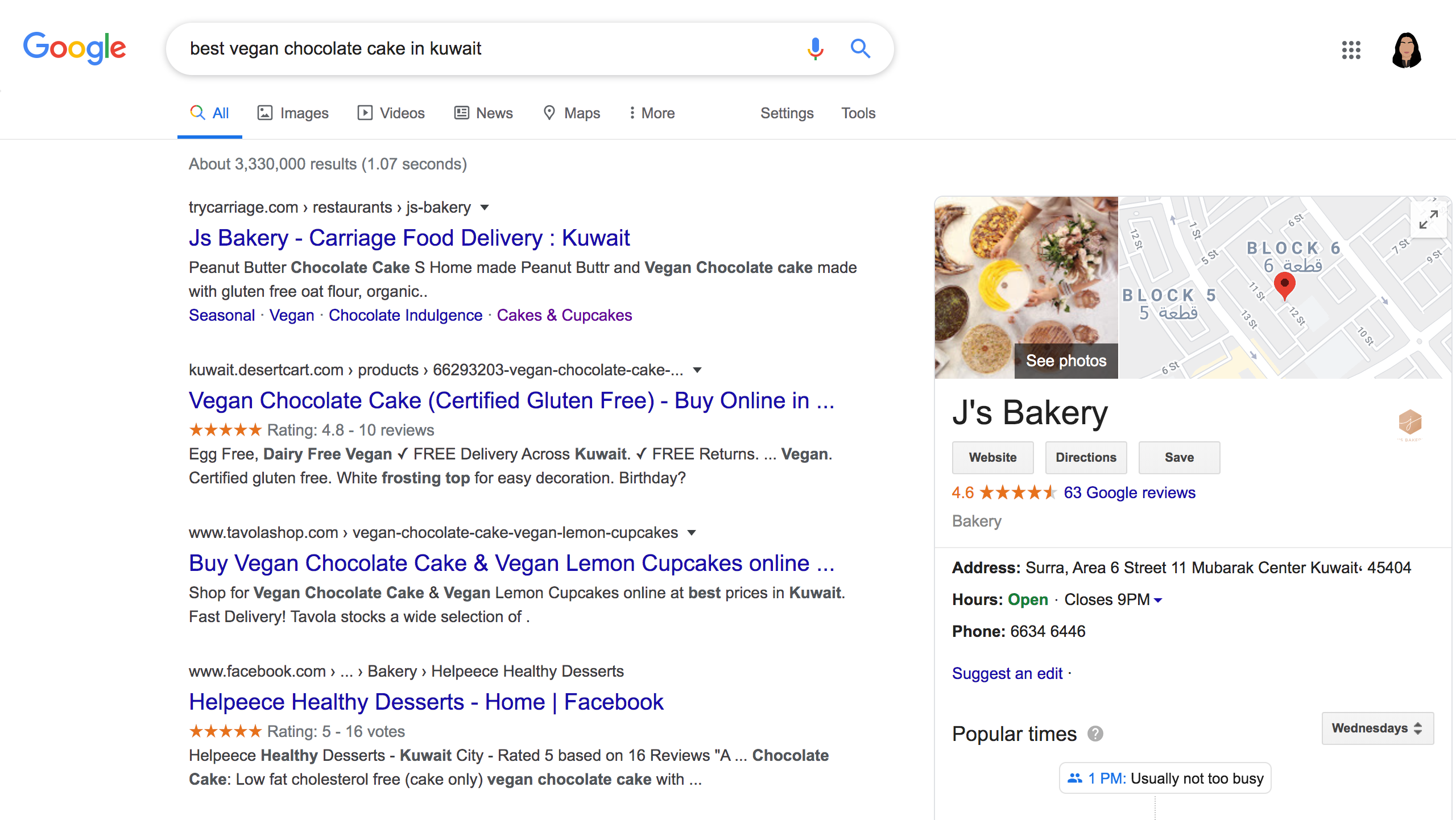A rectangular screenshot from an internet browser displays a Google search results page for "Best Vegan Chocolate Cake in Kuwait." The long side of the rectangle runs from left to right. At the very top of the screenshot, the Google logo is positioned on the far left. Next to it, centrally positioned, is an oblong, white search box outlined in gray, containing the search query. On the far right of the search box are a microphone icon and a magnifying glass (search) icon. 

Outside the search box on the far right, there's a grid icon representing Google's apps, and an icon symbolizing the logged-in user's profile. Below the search box, there are various filter options listed: "All," "Images," "Videos," "News," "Maps," "More," followed by "Settings" and "Tools." The "All" filter is highlighted in blue and underlined, indicating its active status. 

A thin gray line separates this header section from the search results below. The results show that there are approximately 3,330,000 search results found within 1.07 seconds. The visible portion includes four main results on the left:
1. Jay's Bakery
2. Carriage Food Delivery, Kuwait
3. Vegan Chocolate Cake
4. A listing for buying Vegan Chocolate Cake and Vegan Lemon Cupcakes from Peace Healthy Desserts on Facebook.

Each result provides brief details pertinent to the search query for "Best Vegan Chocolate Cake in Kuwait."